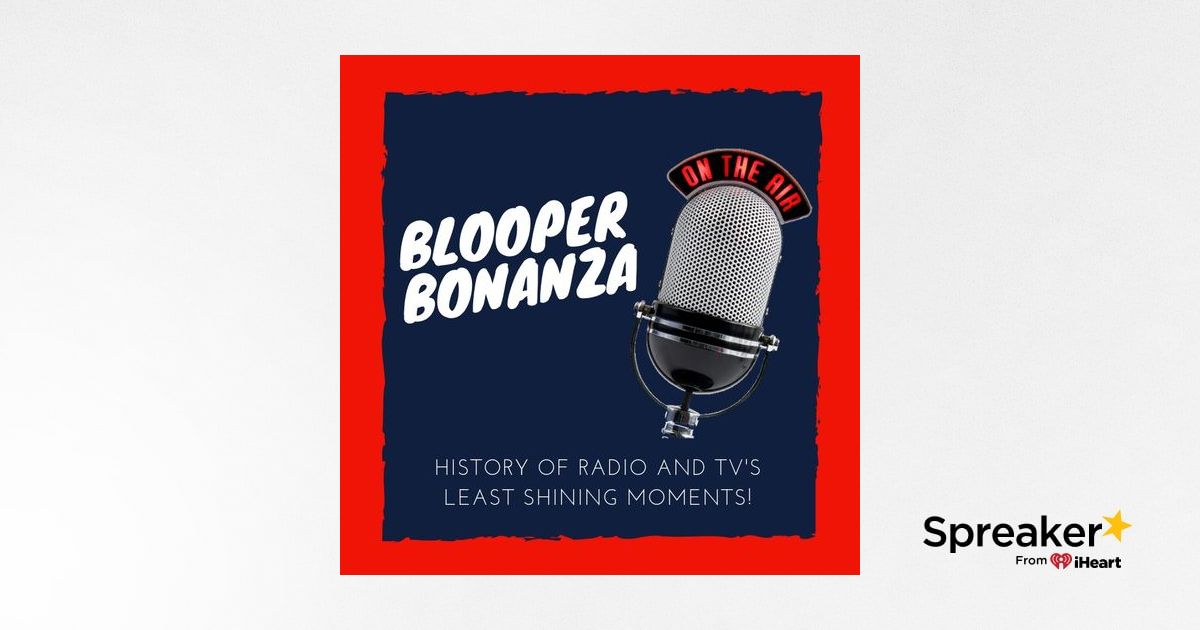This is an advertisement with a red and black square frame, featuring a thick red border and a black outline. At the bottom right, it displays "Spreaker" followed by a star and "From iHeart" in black letters. Within the frame, there is an old-fashioned microphone with a black base and chrome detailing. The microphone displays "On The Air" in neon red letters at the top. To the left of the microphone, in bold white letters, it says "Blooper Bonanza." Below this, in smaller white text, it reads "History of Radio and TV's Less Shiny Moments!" The background of the advertisement is dark blue, giving a stark contrast to the bright and bold elements used in the design.